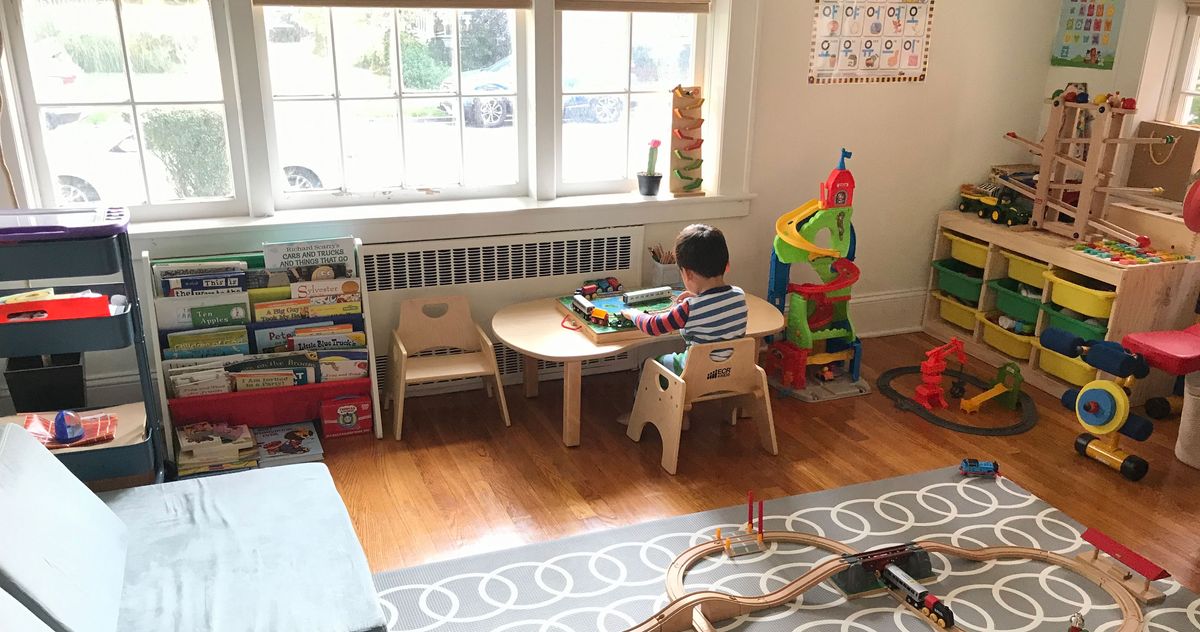The image depicts a vibrant children's play area, likely part of a classroom or daycare center, featuring a rich mix of toys and furniture tailored for young kids. Dominating the scene is a gray carpet sprawled over wooden plank flooring, adorned with a car or train track set up. To the left, a couch provides a cozy seating area. In the middle of the room stands a little boy, his back facing the viewer, engrossed in playing with a train set or cars on a small wooden table and chair. Surrounding him are various educational and playful elements: a magazine rack, wooden blocks, trucks, and other wooden toys. 

In the background, a large window lets in natural light, revealing parked cars outside. Opposite the window, a series of deep shelving units with colored trays (three yellow, three green, and another three yellow), offer ample storage for more toys and supplies. These shelves are topped with a rolling wooden toy that lets balls cascade from one level to another. The walls display cheerful posters, enhancing the child-friendly ambiance. Additional interconnected wooden structures and various other toys are scattered across the floor, making the room a bustling hub of activity and imagination ideal for any imaginative play or early learning environment.